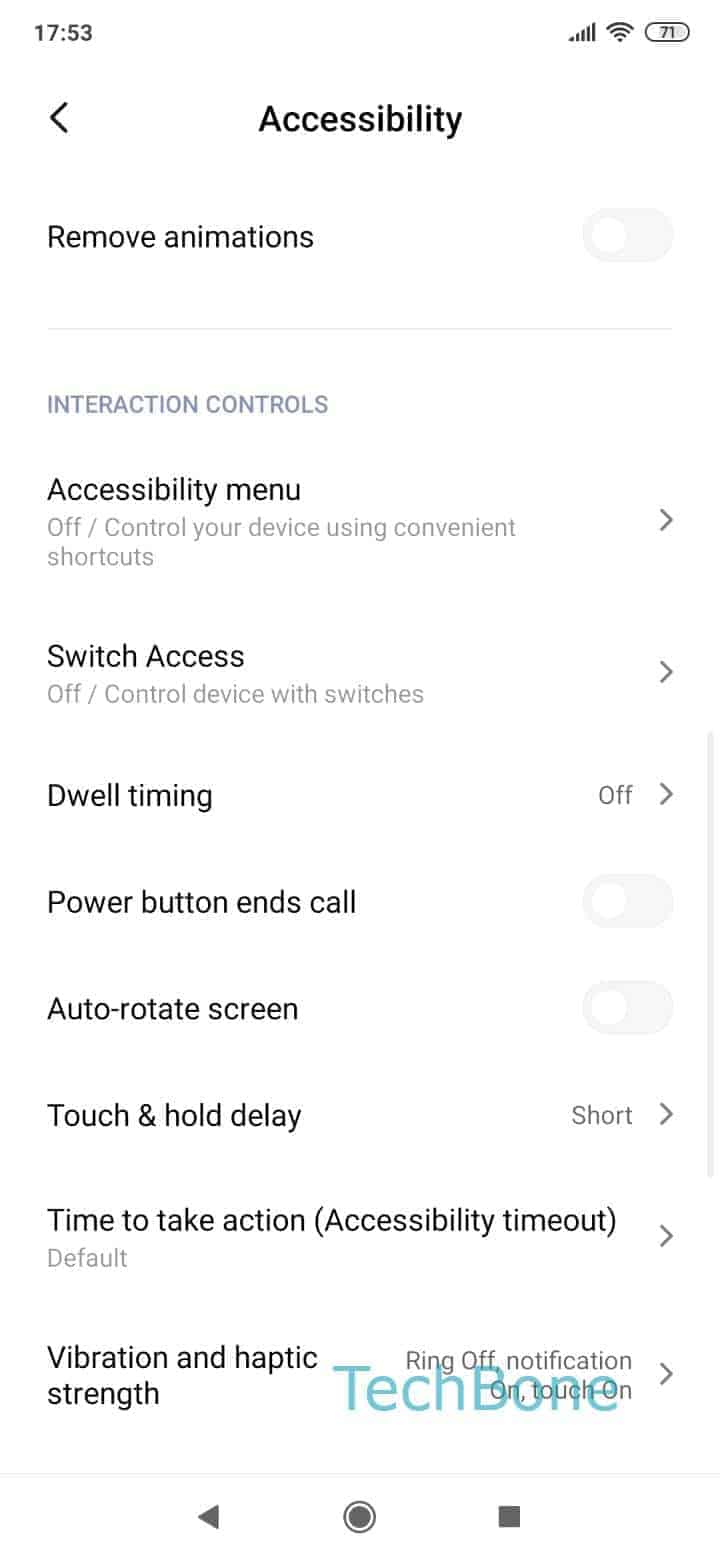The image displays a smartphone screen showcasing the "Accessibility" settings menu. At the top left corner, the time is displayed in military format as 17:53. To the right, the battery icon shows a charge level of 71% with a Wi-Fi signal icon to its left, indicating a connected network, and full bars for phone signal strength.

The main header in the center reads "Accessibility" with a back arrow to navigate to the previous screen. Below the header, there is a slide toggle switch for "Remove animations," which is currently turned off and positioned to the left.

The next section is labeled "INTERACTION CONTROLS" in gray uppercase letters. Below this, "Accessibility Menu" is listed with a description: "Control your device using convenient shortcuts." There's a right arrow indicating that this option can be selected for more details. 

Following this, "Switch Access" is mentioned, which is also off, with a right arrow to further configure this feature. The screen further lists "Power button ends call," currently toggled off to the left, and "Auto-rotate screen," also switched off.

At the bottom, the "Touch and hold delay" is set to short, with a right arrow allowing the time duration to be changed. "Time to take action" and "Vibration & haptic strength" settings follow, with the latter showing "Ring off" and "Notification off." An overlay of blue text partially covers this area, reading "Tech Big Bone" in large font.